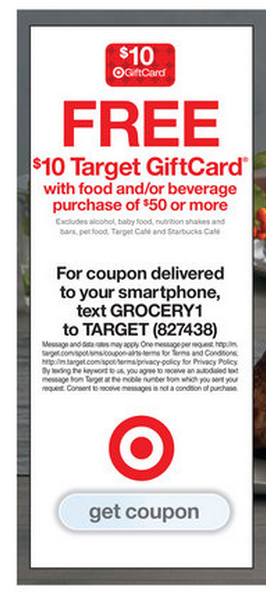The image is a vertically oriented advertisement, roughly three to four times taller than it is wide. It has a narrow gray border, constituting about 5% of the dimensions on the top and bottom, and less than 10% on the sides. Behind the text, faint hints of red, white, and green—the latter possibly representing grass—are visible. This forms the backdrop of the ad.

In the center of the advertisement is a bold white background featuring the distinctive Target branding. At the top is a prominent, red-colored Target gift card graphic, labeled "$10 Gift Card." Directly below this graphic is large, eye-catching red text that simply states "FREE." 

Underneath the word "FREE," in smaller but still significant text taking up about a third of the ad's height, are the words "$10 Target Gift Card." The message continues below that, occupying approximately half the remaining height, and specifies "with food and/or beverage purchase of $50 or more."

Further down, the advertisement lists exclusions in small, gray text: "Foods, alcohol, baby food, nutrition shakes and bars, pet food, Target cards, and Starbucks card." This section is difficult to read due to its size and color.

At the bottom, there is a black text instruction that reads: "For coupon delivered to your smartphone, text Grocery1 to 827438 (Target)." 

Overall, the advertisement is vivid and immediately identifiable as belonging to Target, offering a clear and enticing promotion for customers.